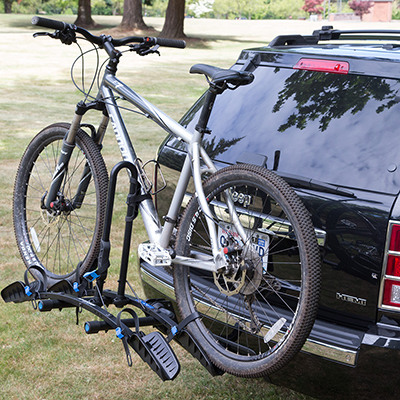The image depicts the back of an old-style, black Jeep SUV, parked on a grassy field under the bright sun. The Jeep features a noticeable Jeep logo centrally placed on the top portion of the bottom half of the hatch door, with a small HEMI badge on the bottom right of the hatch. The upper part of the hatch door consists of angled glass, complete with a windshield wiper at the top. The tail lights are framed in chrome, adding a sleek touch. Mounted on the back of the Jeep is a black metal bike rack designed to hold two bikes, though only one white and gray mountain bike with tread-heavy tires is currently secured in place. The grassy field appears slightly yellowish-green, hinting at the outdoor and possibly park-like setting. The background features several tree trunks providing shade, adding to the serene, outdoor atmosphere of the scene.